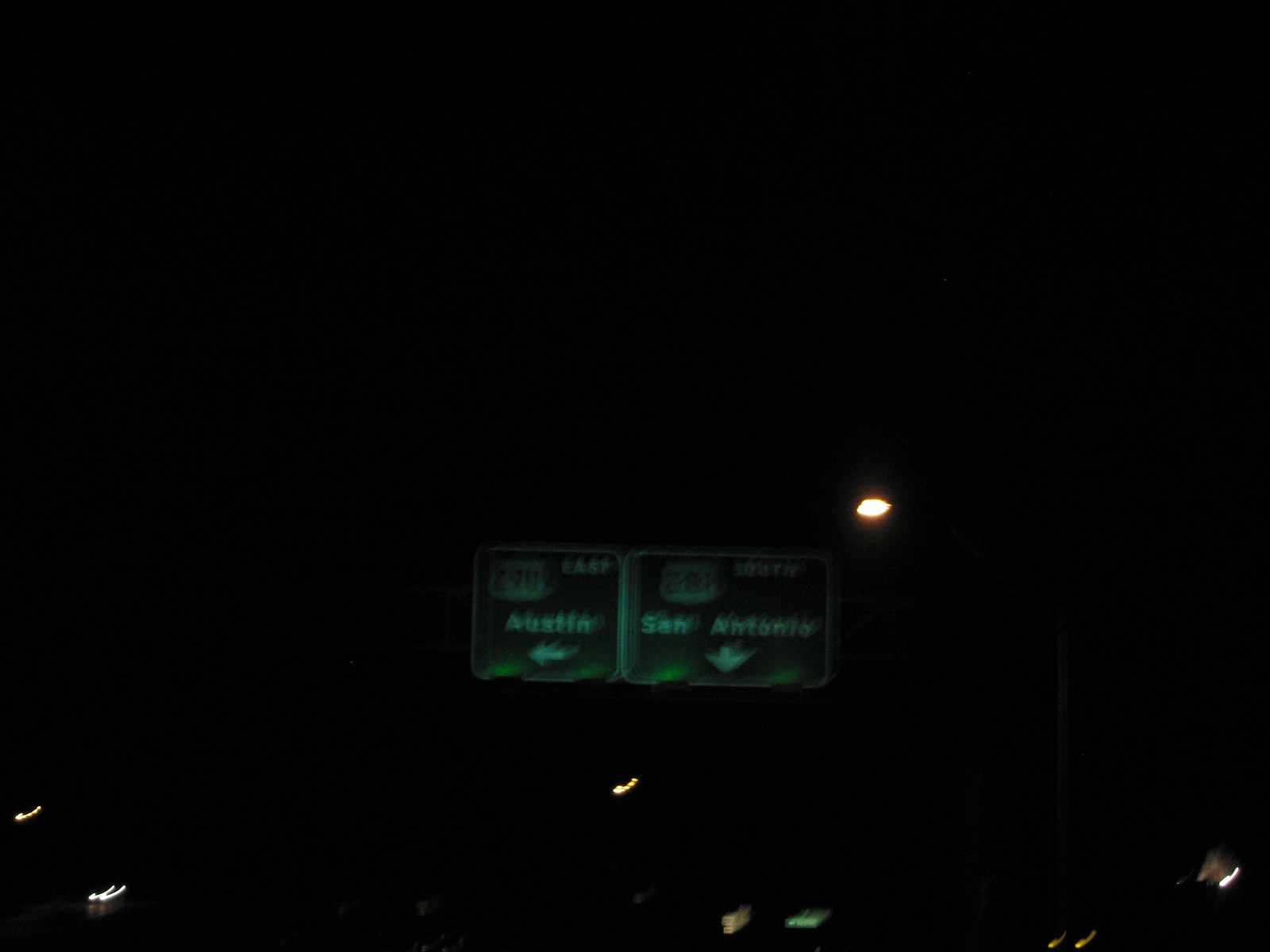A grainy nighttime photograph captures a pair of green freeway signs illuminated by street lights. The image is predominantly dark, almost black, with the signs at the center bottom. Both signs are mounted on a post with a lamp, casting light upon them. The left sign indicates "290 East Austin" with a left-pointing arrow and is adorned with two small lights. The right sign displays the route number "281" inside a shield emblem, with the word "South" adjacent to it, followed by "San Antonio" and a downward-pointing arrow. The image quality is low, resulting in a blurry and pixelated appearance. Scattered throughout the darkness, specks and streaks of light hint at moving vehicles, adding to the ethereal and chaotic ambiance of the scene.